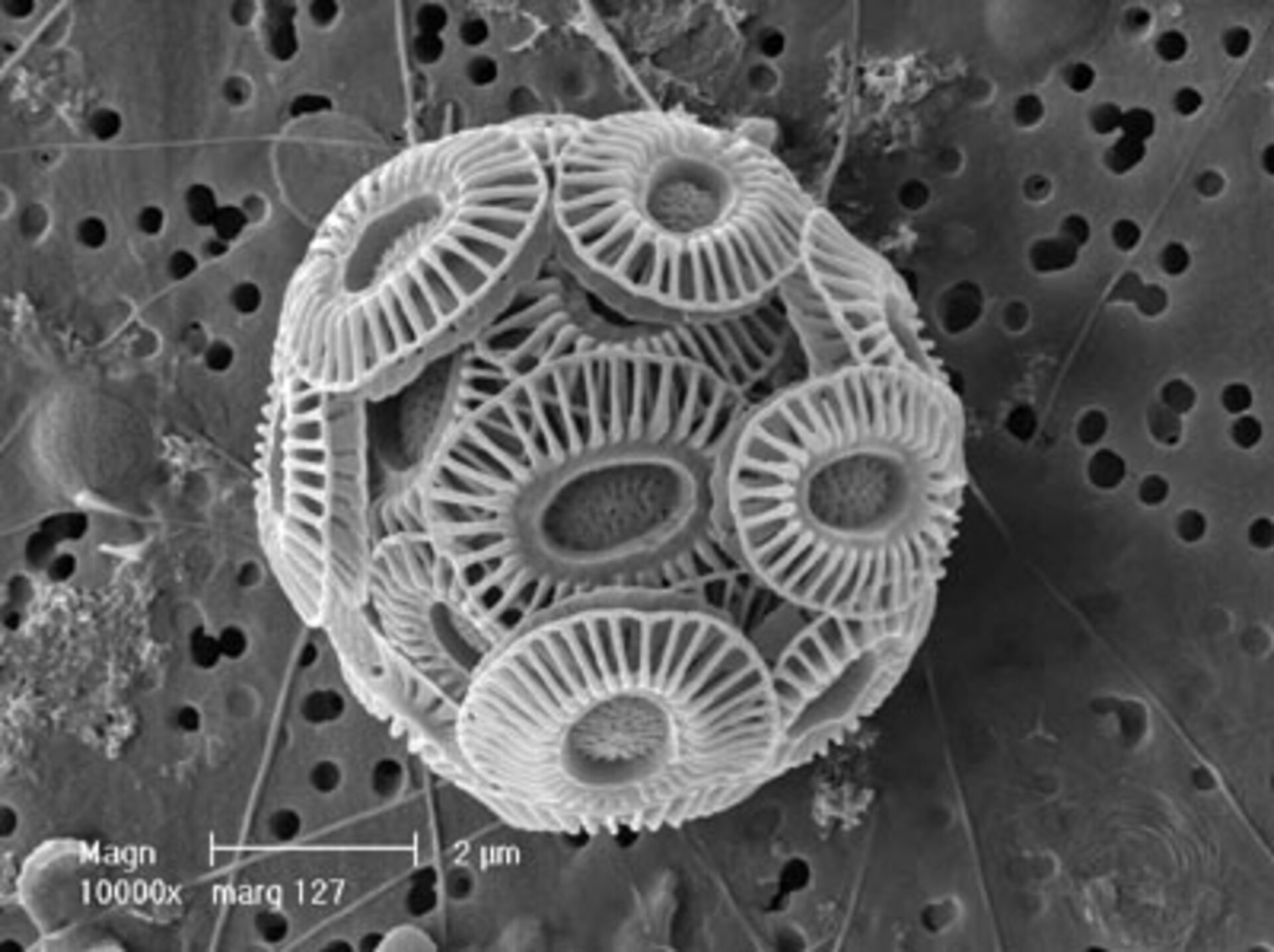This black and white microscopic image captures a detailed view of a round, cell-like structure with oval pieces overlapping one another, resembling a volleyball. Each oval has a ring in the center with white strands radiating outward, all interconnected by a solid white line. The background is covered in a porous material with variously spaced holes, some solitary and others clustered together, featuring ribbed or veined patterns throughout. In the bottom left corner, text reads "MAGN 10,000X" above a meter line marked "2 µm" and the notation "Marge 127." The entire scene presents shades of black, white, and gray, meticulously showcasing the microscopic world.